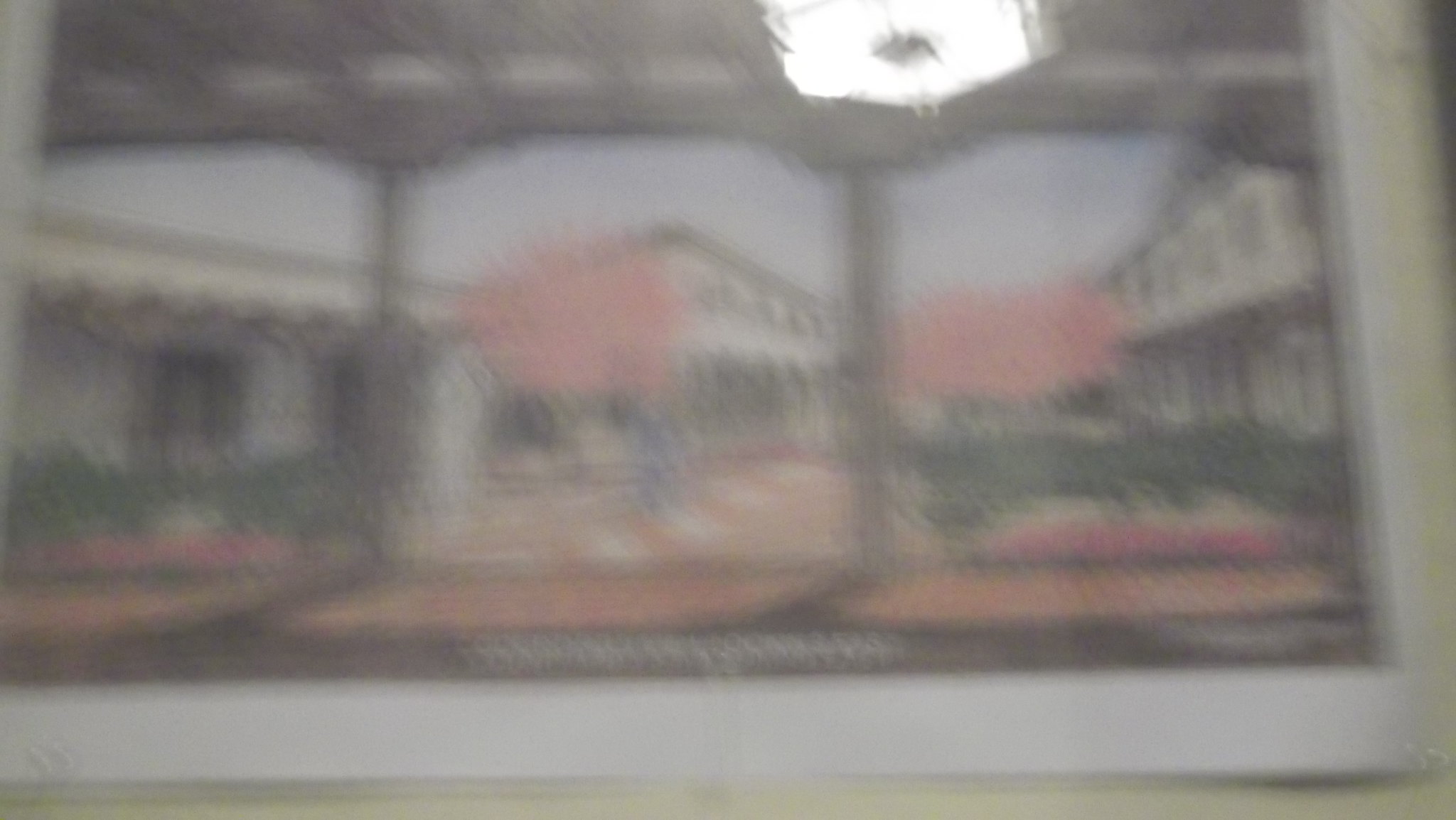This image is highly blurred and depicts a framed photograph lying on what seems to be an eggshell white tabletop. The photograph itself is divided into three distinct segments that create a cohesive scene, resembling a row of hacienda-style buildings. The buildings are tan with cobblestone fronts, black windows, and black roofs. Below the frame, a portion of the white picture border is visible, and towards the top right, there's a bright ceiling light fixture creating a glare. The background includes a gray sky and some trees, with one prominently displaying reddish blossoms. The overall structure and details are faint and indistinct due to the blurriness of the image.